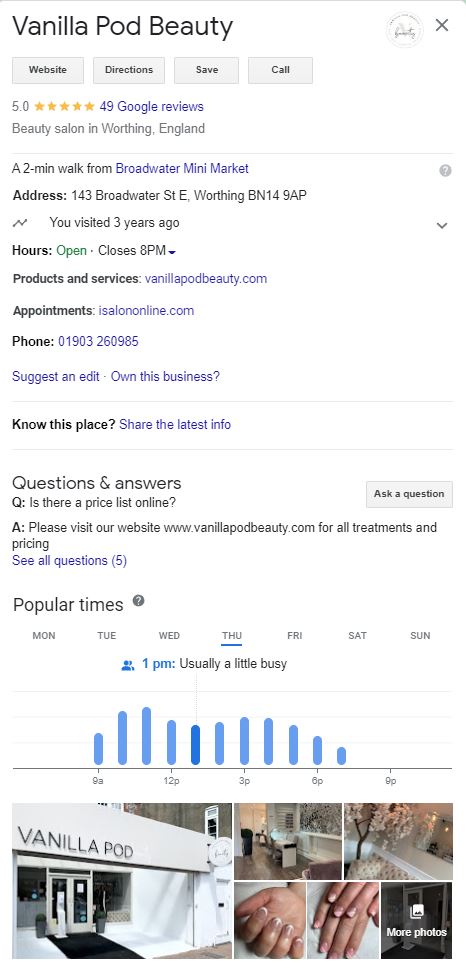Here is a cleaned-up and detailed descriptive caption for the provided image:

---

This image is a Google Business entry for "VanillaPodBeauty," prominently displayed at the top left in bold black letters. Four category buttons appear below the business name: "Website," "Directions," "Save," and "Call." VanillaPodBeauty boasts an impressive rating of 5.0 stars, illustrated by five yellow stars, alongside a clickable link to 49 Google reviews. Categorized under "beauty salon," this business is located in Worthing, England, just a two-minute walk from the hyperlinked Broadwater Mini Market.

The business address is displayed, with a note indicating a visit three years ago. Beneath this, the entry includes categories for "Hours," "Products and Services," "Appointments," and "Phone." Options for "Suggest an edit" and "Own this business" are hyperlinked.

Further down, users are prompted with "Know this place?" and a hyperlink inviting them to "Share the latest info." At the bottom of the page, a line graph illustrates the popular times of day, indicating crowd levels, followed by thumbnails showcasing the business and its products.